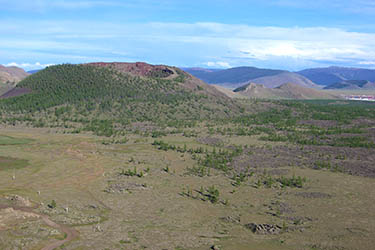The image features a breathtaking bird's-eye view of a vast, serene landscape dominated by expansive hills and large mountains stretching all the way to the horizon. The foreground presents a green meadow interspersed with patches of brown dirt and sparse greenery, perhaps moss or weeds. In the background, a large imposing mountain, which appears to have a crater-like formation at its center, rises prominently. This mountain is surrounded by lush greenery that includes a mix of trees and bushes. Hills and smaller peaks are also visible, creating a layered look that extends into the distance, giving a sense of endless terrain. The sky above is a brilliant blue, dotted with an array of fluffy white clouds in varying shades. The overall image captures the tranquil beauty and vastness of nature from a high vantage point, possibly taken from another mountain, a drone, or a helicopter.